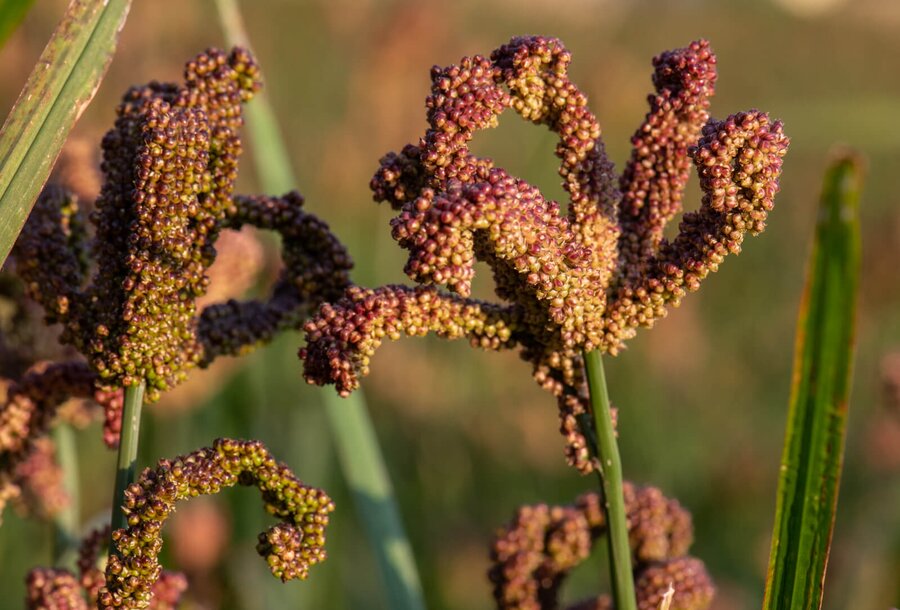The digital photograph features a close-up of clustered flower buds or berries with a rich, rosy red hue intermixed with some brown tones. These buds or berries are densely packed on two prominent stems that appear short and wide. Surrounding these stems are vibrant green blades of grass and stems, which stand out clearly against a blurry background. The top of each plant is covered in small seeds, resembling tiny eggs or detailed textures, reminiscent of a petaled rose where the petals would be. The overall color palette includes shades of light green, yellow, purple, black, and gray, but the most striking elements are the red and green hues of the plant structures. No visible text is present in the image, and the entire scene suggests an intimate zoomed-in perspective of a rich botanical environment.